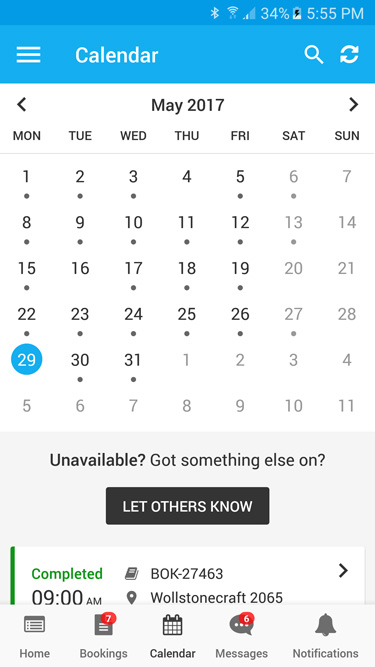Screenshot of an Android mobile device displaying the calendar view for May 2017. The interface features a monthly calendar with the days of the week listed along the top, and individual days arranged in a grid format. Each day includes a small dot underneath it, potentially denoting appointments or events.

At the bottom of the screen, there is a section labeled "Completed" which details a specific booking with the reference BOK 27463, scheduled for 9:00 a.m. in Wallen Stonecraft 2065. A message is displayed indicating that the user is not available and prompts them to inform others by clicking the "LET OTHERS KNOW" button, highlighted within a black clickable square.

The navigation bar at the bottom of the screen includes icons for bookings, the calendar, messages, and notifications. Each icon has a small red badge, serving as a notification indicator. The bookings icon shows seven new notifications, while the messages icon shows six new notifications.